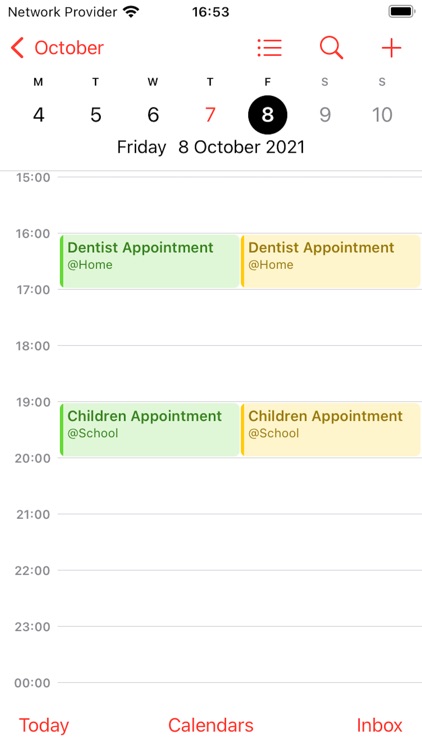A detailed screenshot of a mobile device calendar is displayed. At the very top of the screen, icons indicate the network provider, the current time (16:53), and the battery status. Just below, the screen displays the month as October, alongside icons for the menu, search function, and a plus symbol to add events to the calendar.

The days of the week are marked by single-letter abbreviations (M, T, W, T, F, S), corresponding to Monday through Saturday. The dates for these days are 4, 5, 6, 7, 8, 9, and 10, with the 8th highlighted in a black circle with white text.

Indicating that the date is significant, it is listed below as "Friday, 8 October 2021" in black text. The main portion of the screenshot details the day's schedule, displaying time slots from morning to evening. Notably included are:

1. A "Dentist appointment" listed at home, spanning from 16:00 to 17:00 (4 PM to 5 PM), with two listings in different colors—green and yellow.
2. A "Children appointment" at school, overlapping between 19:00 and 22:00 (7 PM to 10 PM), also marked with green and yellow entries.

The bottom section of the screen, with red text, provides navigation options labeled "Today," "Calendars," and "Inbox" against a white background, ensuring easy user interface navigation.